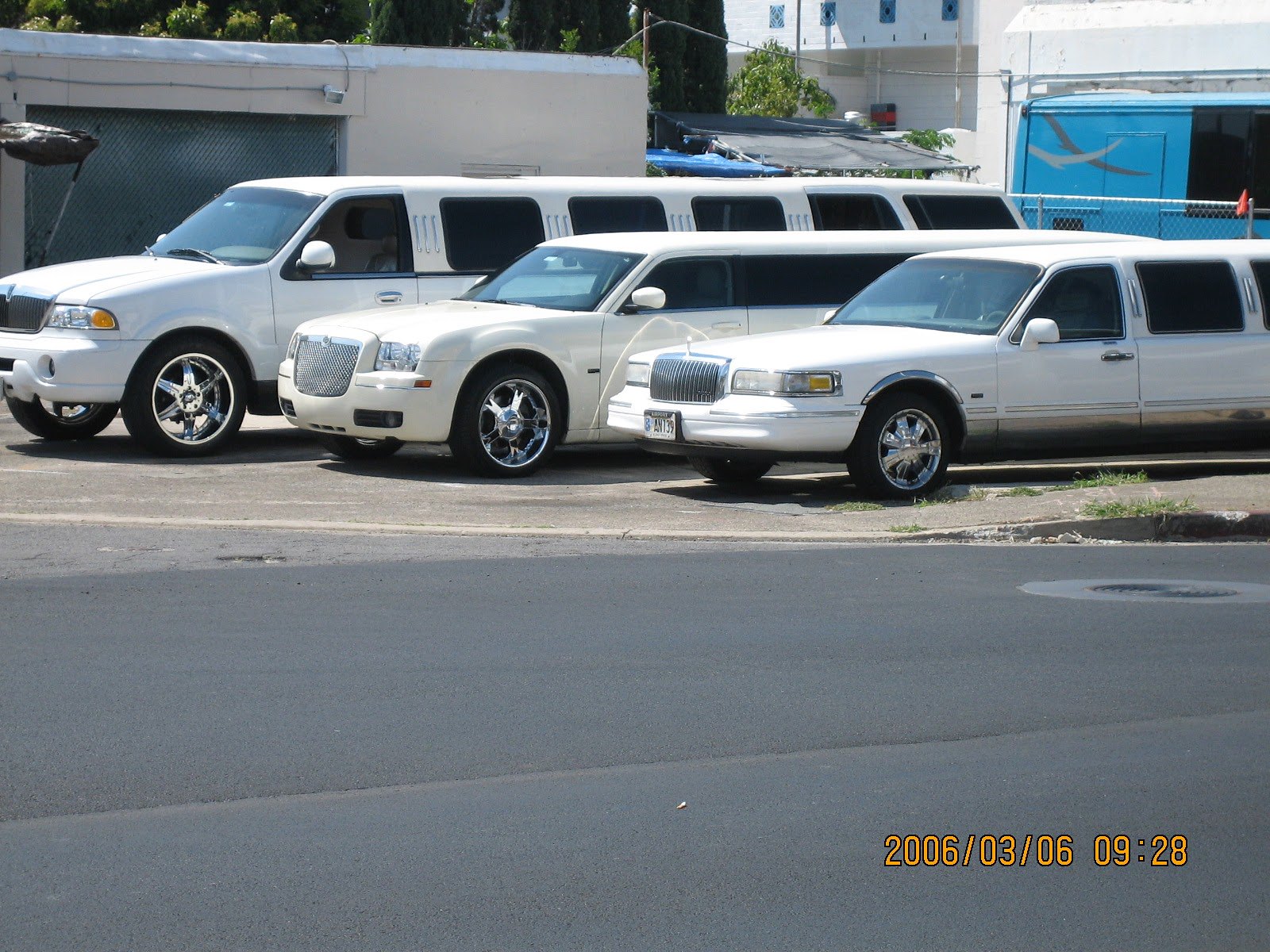This landscape-oriented, full-color photograph, taken at 9:28 AM in 2006, captures three white limousines parked side by side in a concrete parking lot. The limousines, each of different makes, showcase tinted black windows and silver grilles. The foremost limousine resembles an SUV with five rows of seats, the middle one appears to be a Rolls Royce, and the last one is a standard American-made stretch limo. Black tires with silver rims complete their sleek, elongated bodies. A blue utility van and a low beige-gray building with white trim are visible in the background. On the bottom right of the image, yellow writing displays the date as "2006-03-06." Surrounding the scene are trees and two houses—one on the left with a white facade and a silver door, and another accompanied by a black object with a white stand. The asphalt road runs in front of the parked limousines.